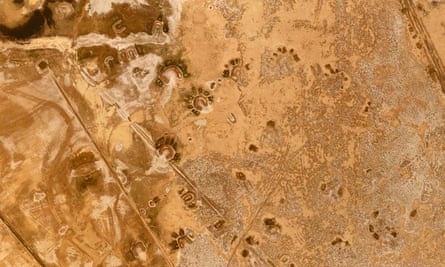This image is a detailed aerial photograph capturing a vast, arid landscape characterized by muted, marbleized shades of pink terracotta, brown, tan, taupe, and gray. The composition, somewhat abstract, mimics the intricate patterns of granite with blotchy, layered colors and a mixture of circular and linear strokes, giving it a three-dimensional quality. Sparse and barren, the region appears devoid of visible structures, animals, or humans, adding to the sense of isolation and calm. Dotted with small white patches that could be snow, the terrain may suggest a colder environment. The subtle presence of what might resemble footprints or sets of trees from this altitude enhances the depth and intrigue of the scene. This rectangular, frameless image is relaxing to observe, invoking a sense of quiet desolation.